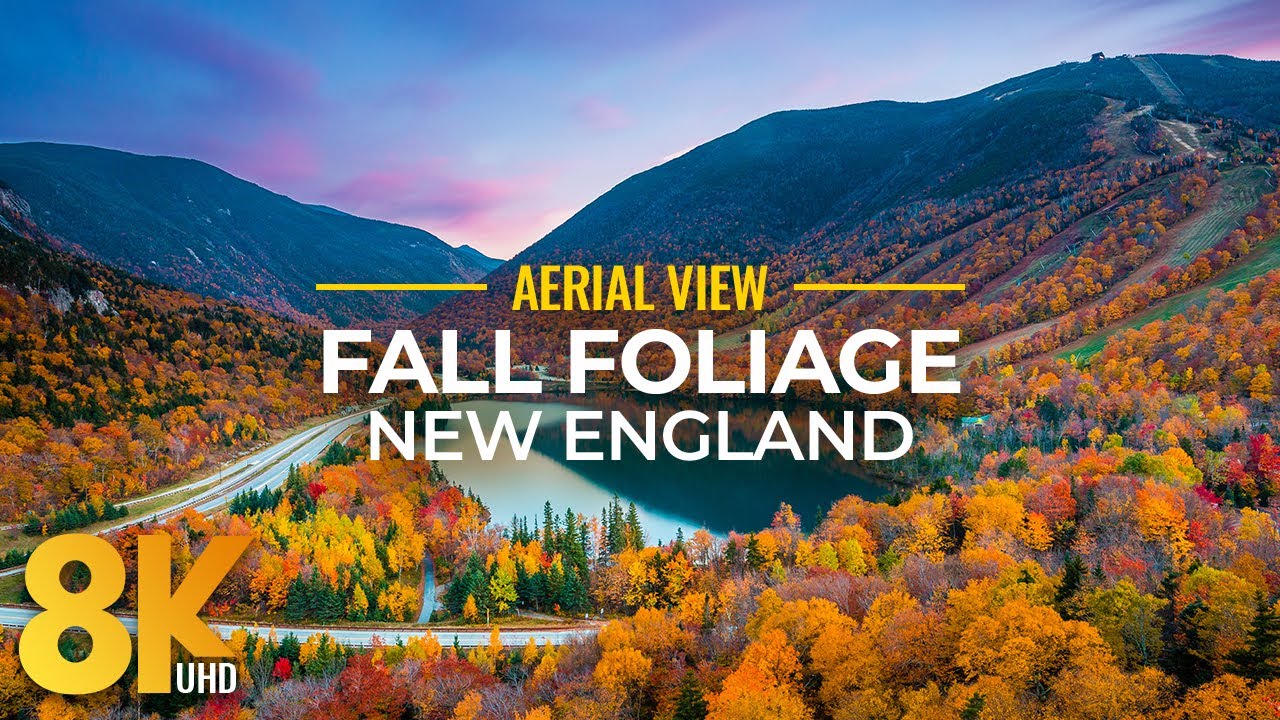This image is a stunning and colorful aerial landscape, possibly a book cover or a large postcard, capturing the breathtaking fall foliage of New England. It features a picturesque valley framed by rolling hills adorned with trees in vivid autumn hues of yellow, orange, red, and green. A small pond or lake and surrounding roads can be observed from this high vantage point. The sky is a magnificent tapestry of sunset colors, ranging from deep blue and purples to bright pink clouds. Dominating the upper portion, the text reads "Aerial View Fall Foliage New England" in bold, standout fonts. Positioned at the bottom left corner is a professional marking, "8K UHD," indicating the high-resolution quality of the image. The overall scene is bathed in the warm glow of late afternoon, enhancing the natural beauty of the landscape.